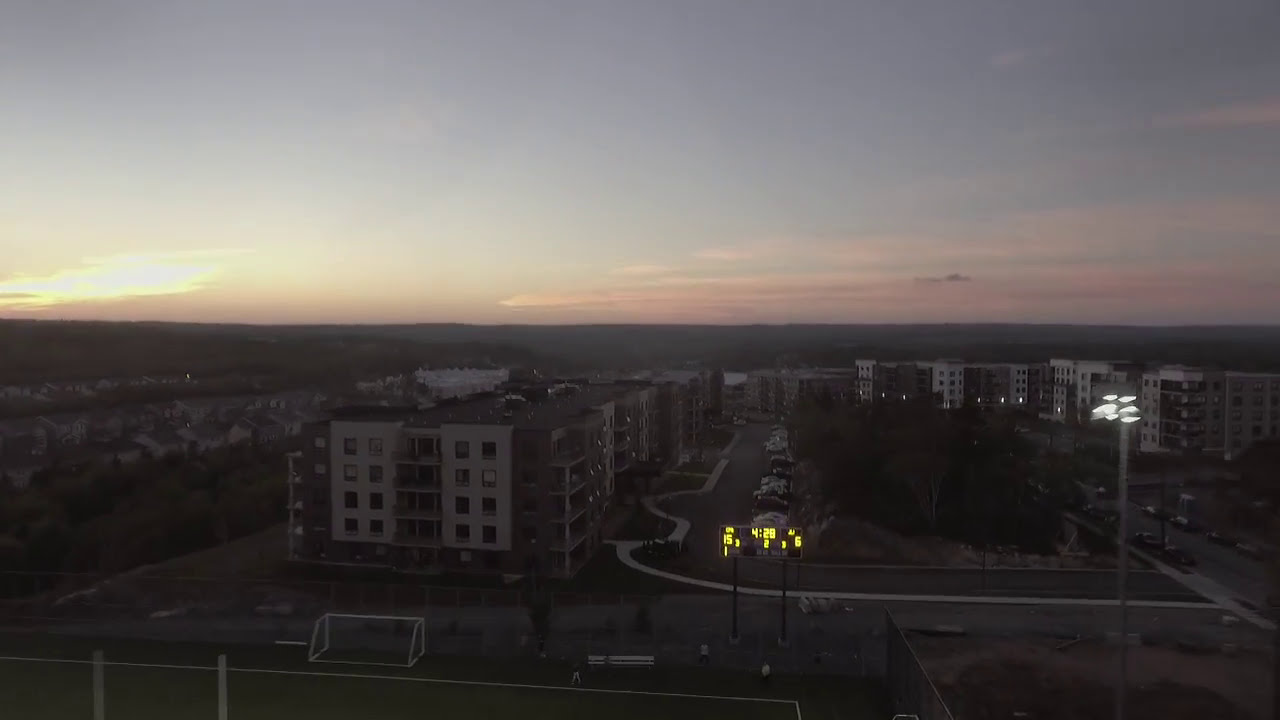An overhead view photograph captures a vibrant neighborhood at sunset, where the fading light casts a unique blend of colors across the scene. The sky transitions from a deep blue to pink and yellow hues around the horizon, evocative of the sun just setting. The majority of the frame is filled with towering gray and white apartment buildings, their windows and balconies clearly visible. The area appears to be a gated community, distinguished by a brightly lit guardhouse at the entrance. 

On the right, a streetlamp is illuminated, casting a soft glow over the surroundings. Below, you can spot parked vehicles along the roads that weave through the neighborhood. To the left, some individual houses dot the landscape, while trees fill the spaces not occupied by buildings and thoroughfares, adding patches of greenery to the scene.

In the foreground, the details of a sports ground come into view, including a prominent goal post and a scoreboard showing the lights, time, and score. The area is devoid of people, contributing to a tranquil atmosphere. Beyond the structures and foliage, the background reveals distant hills, accentuating the picturesque quality of this sunset moment.